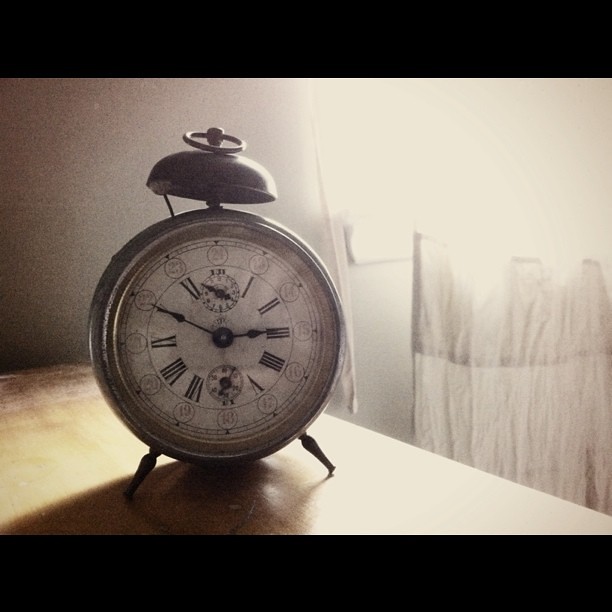This photograph features a vintage-style alarm clock, prominently positioned on a light wooden dresser within a bedroom setting. The clock, crafted from metal, showcases a weathered silver finish accented by spots of rust around its rim, indicative of its age. Its classic round design is topped with a large metallic bell, which serves as the alarm mechanism, and is activated by a small metal hammer protruding from the left side.

The clock face is pristine white and marked with black Roman numerals that denote the hours, while additional numbers encircle the face, further detailing the time. The clock boasts two hands—a longer minute hand and a shorter hour hand—both black and metallic with arrow-shaped tips. Above these is a smaller inset dial likely indicating the seconds.

In the background, a window on the right side hints at the room's layout, complemented by horizontally striped curtains in light and dark gray. The juxtaposition of the old-fashioned clock against the modern bedroom decor offers a charming contrast, drawing attention to the timeless nature of the timepiece.